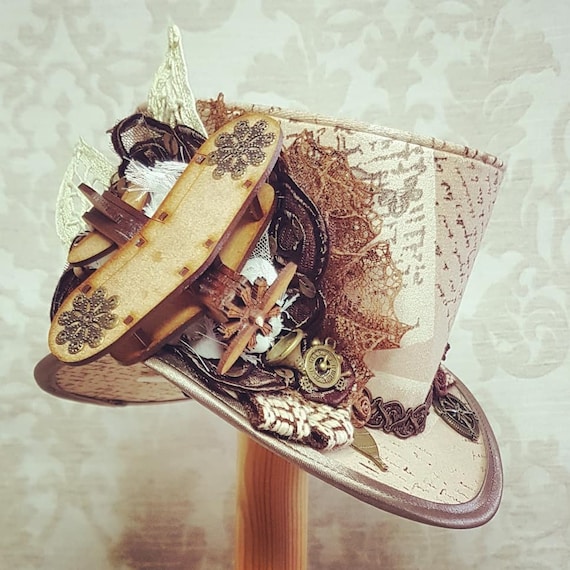The image features a close-up of a customized Mad Hatter-style top hat, prominently displayed against a fancy, floral-patterned wallpaper of off-white and light pastel colors. The hat itself, perched atop a wooden stick or pole, is a striking piece with a beige and light brown color scheme. It sports a brown braided band around the base of its crown, where the crown meets the brim. The top of the hat features old handwriting, resembling a vintage letter or newspaper print.

The brim of the hat is accentuated with a brown fabric trim. On the left side, an elaborate array of decorations includes a mix of reddish, black, and brown fabrics, intertwined with a wooden airplane, complete with a small propeller and snowflake symbols on its wings. Additional accessories like brown lace, a small trumpet, and ribbons in burnt orange, tan, black, and white add to the hat's eclectic charm. The intricate design might suggest a touch of leather spirals and abstract patterns. Overall, the hat evokes a whimsical, old-timey feel, reminiscent of something one might wear to a grandiose event or race.